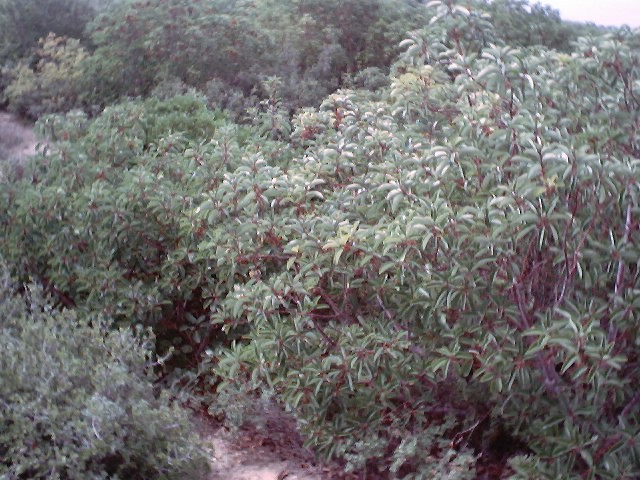The photograph, taken outdoors on a cloudy day, depicts a dense, lush forest scene. In the lower left-hand corner, a narrow, unclean dirt path meanders through underbrush and foliage, curving slightly to the right before disappearing farther back into the trees. The path and the foliage suggest a potentially challenging hike. The center and right side of the image are dominated by thick vegetation, including large green bushes with occasional brown leaves. The trees splay out towards the sky, with their vibrant green canopies contrasting against the white, overcast sky visible in the top right corner. The colors are predominantly greens of varying shades, with the path and dirt providing tans and browns. The path appears to connect through denser foliage in the top left of the image, suggesting continuity for any adventurous hiker willing to navigate the forest. The photograph encapsulates the vibrant and somewhat untamed beauty of nature, embodying the feeling of venturing on a forest trail in the midst of the day.